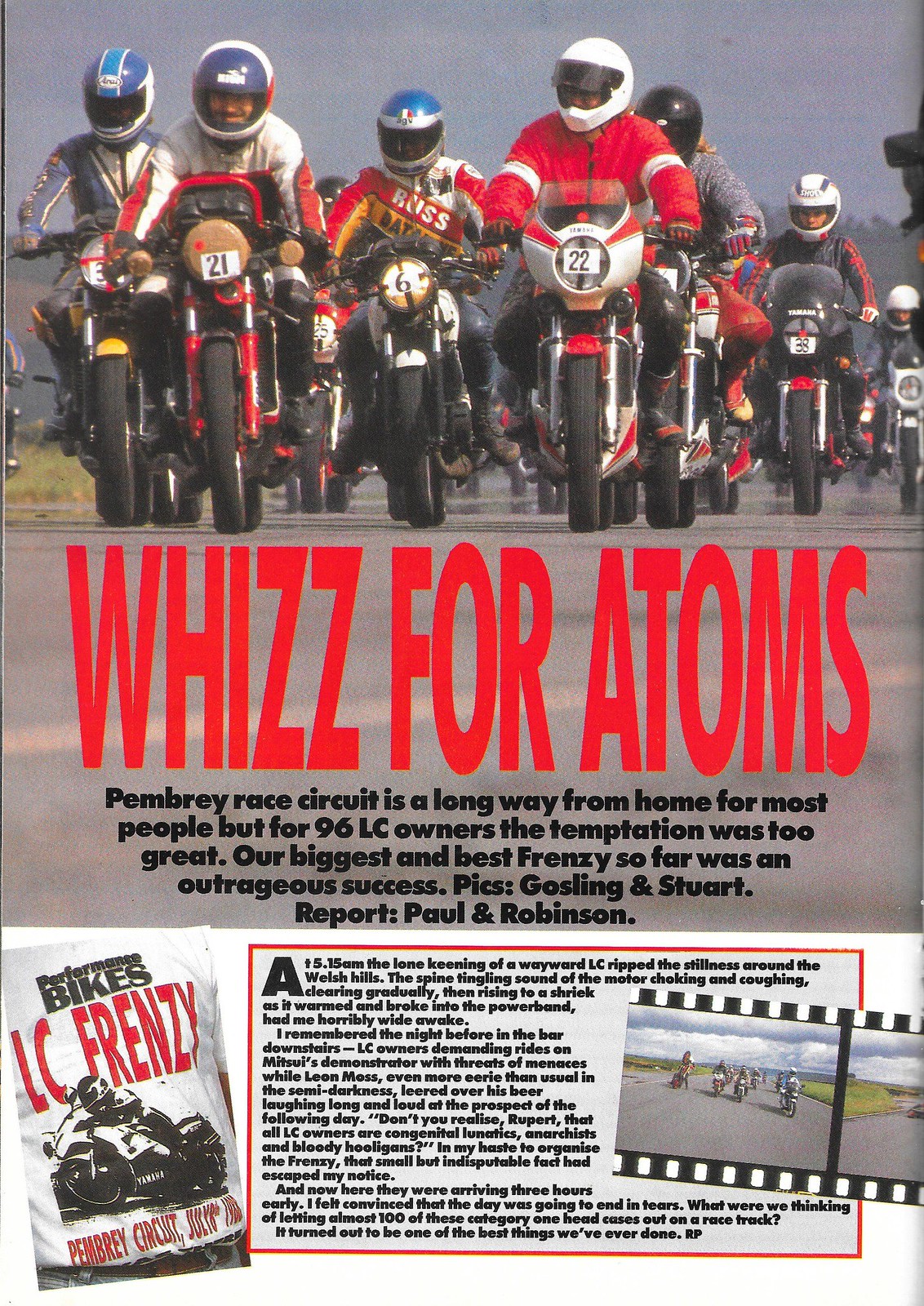The magazine page showcases a vibrant image capturing a thrilling scene of a motorcycle race, featuring several motorcyclists in full racing gear, including helmets in blue, white, and black. Each motorcycle bears a distinct number such as 21, 25, 6, 22, and 38, indicating a competitive event. The motorcyclists are seen speeding on a road, possibly at the Pembrey Race Circuit, which, as the accompanying text suggests, is far from home for most participants. Despite the distance, 96 LC owners couldn't resist the call, resulting in the biggest and most successful frenzy yet. The bold red text "Whiz for Adams" stands out prominently above the photograph. Additional content includes reports by Paul and Robinson, with Gosling and Stewart providing photographic evidence of the event. The narrative vividly describes the early morning commotion at 5:15am, as the spine-tingling sound of an LC motorcycle broke the quiet of the Welsh hills, warming up to a shriek. The magazine page also references a lively night before at the bar, setting the stage for the high-energy event that followed, filled with eager LC owners and their spirited antics. A black ink drawing of a motorcyclist adds to the page's dynamic layout, emphasizing the frenzied and anarchic spirit of the event.